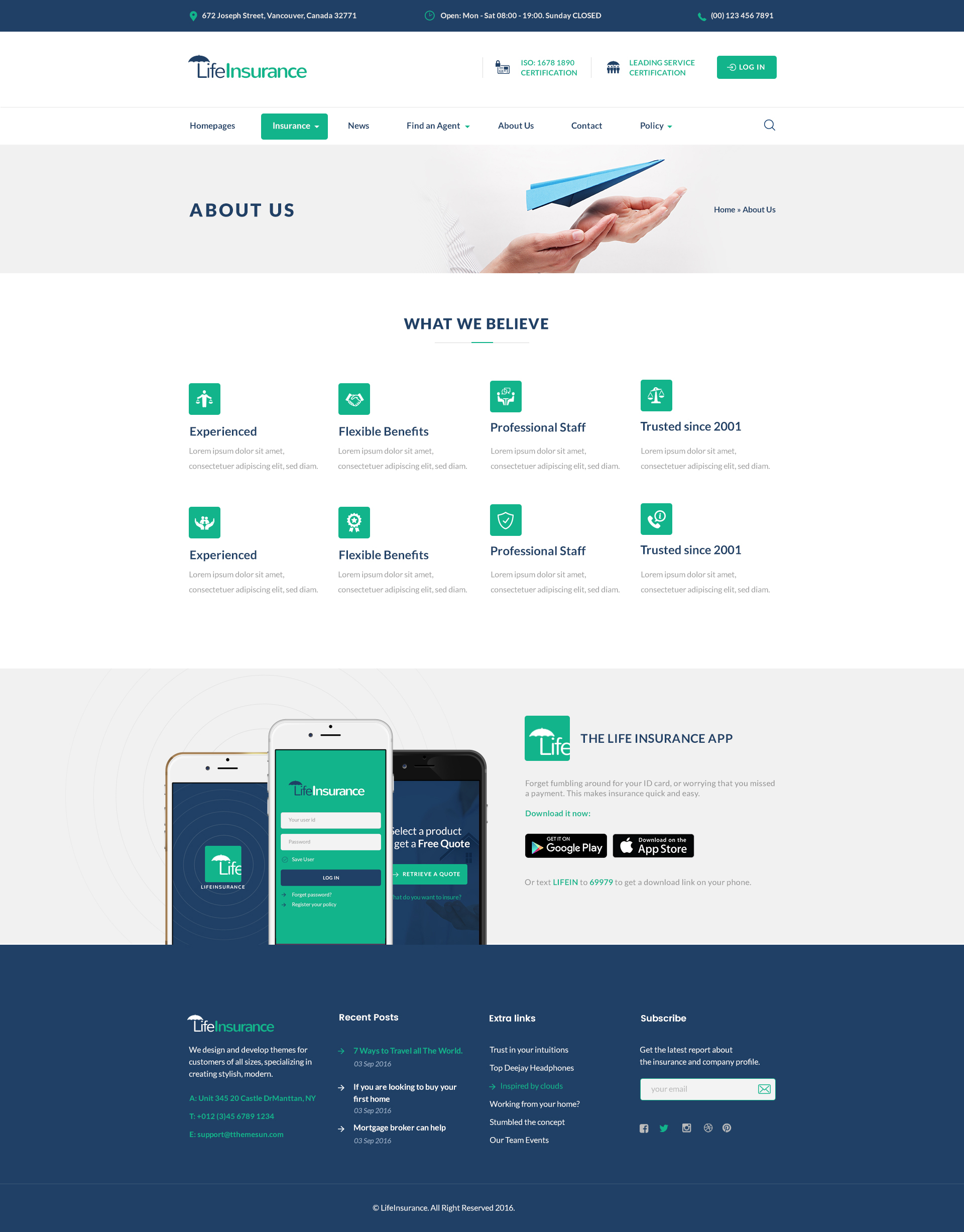This image showcases a professionally designed website, which appears to be a template available for purchase or possibly a live site. The website has a blue header bar at the top, displaying a physical address: 672 Joseph Street, Vancouver, Canada, 32771. To the right of the address is a clock icon indicating the operating hours: open from Monday to Saturday, 8:00 AM to 7:00 PM, with closures on Sundays. Further to the right is the phone number: 001234567891.

Below the header on the left side is a logo featuring the text "Life Insurance" where "Insurance" is in green and "Life" is topped with an umbrella over the letter "L." Adjacent to the logo is a lead certification icon and a login button. 

A navigation menu is situated below the header, with options for "Home," "Pages," and "Insurance," the latter being highlighted in green. Additional menu items include "News," "Find an Agent," "About Us," "Contact," and "Policy."

The main focus of the page is the "About Us" section, presented with an image of an upraised hand holding a blue paper airplane. Following the "What We Believe" section, the page features eight icons with headers such as "Experience," "Flexible Benefits," "Professional Staff," "Trusted Since 2001," and "Experience" (repeated), among others. The section also includes images of three smartphones showcasing how the website appears on mobile devices.

On the right side, there are options to download the insurance app from Google Play and the App Store. The footer at the bottom of the webpage provides links to posts, social media icons, a subscribe button, and contact information.